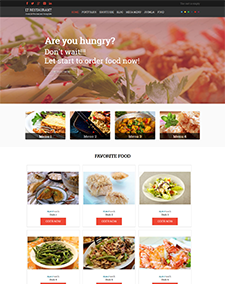The image displays a web page open to an online food ordering service. Prominently featured at the top is a bold, inviting message: "Are you hungry? Don't wait. Let's start to order food now." The design of the website exudes sophistication, suggesting a higher-end dining experience. In the background, luxurious floral arrangements contribute to the elegant aesthetic, while the main focus remains on the diverse food offerings.

At the top section of the webpage, there are four distinctive food dishes depicted. Though it's challenging to identify each one precisely, the variety includes what appears to be a Chinese stir-fry and a possible dessert among the selection. 

Below this, a section titled "Favorite Foods" showcases six different items. These include a pan-seared meat dish, a cake topped with crumbles, and a fresh salad. Additionally, there is a dish featuring green beans or other vegetables, a middle casserole, and a rightmost entry that seems to be a seafood dish, although its exact nature is ambiguous.

The layout suggests that users can scroll down to explore more offerings beyond what is immediately visible, implying a comprehensive menu. The "Favorite Foods" could either represent popular choices among all users or personalized favorites based on previous orders. Overall, the webpage invites users to easily browse and order a variety of appealing dishes, all from the comfort of their device.